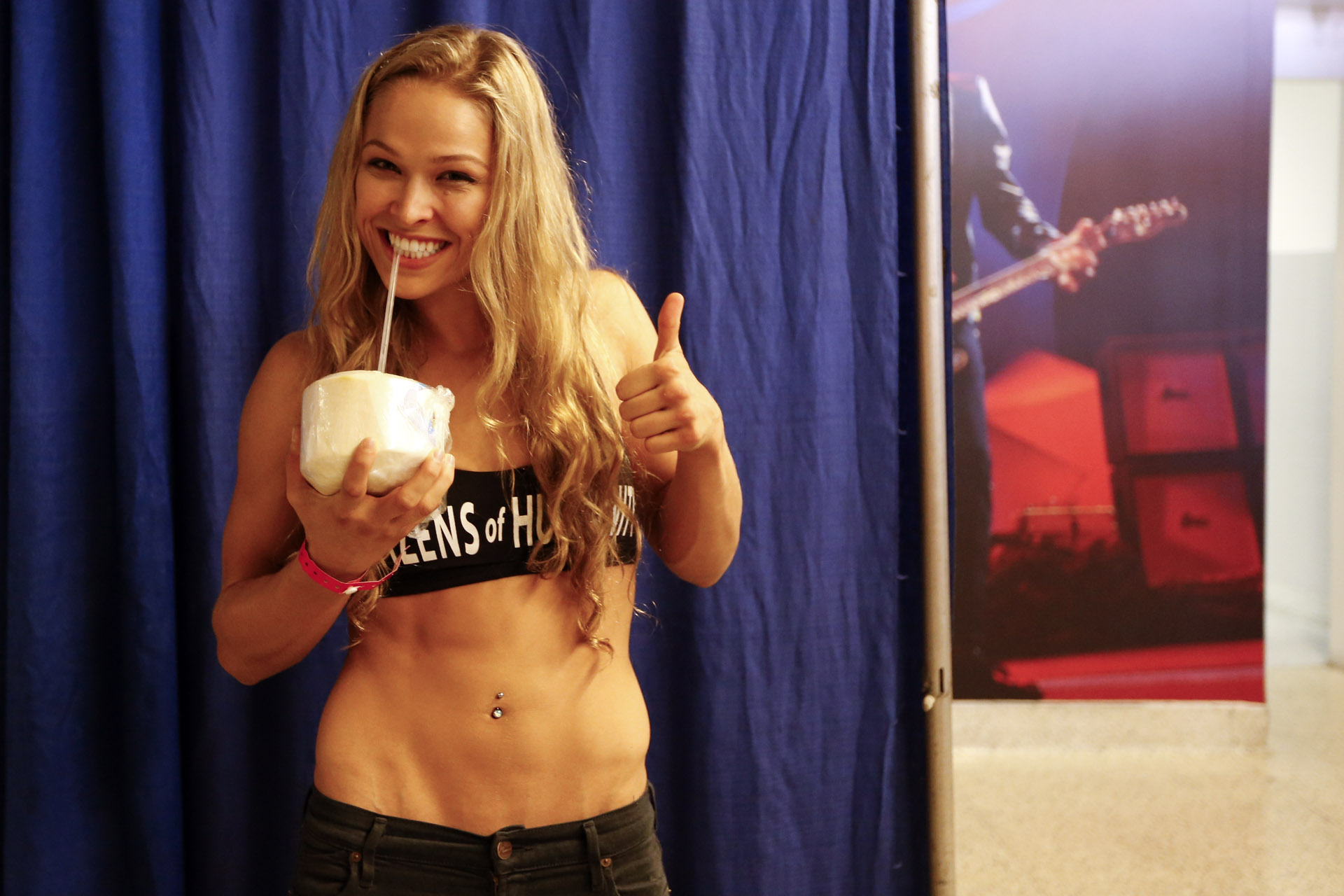The photograph captures a fit young woman with long blonde hair that cascades down to her belly button, standing against a dark blue curtain that covers most of the backdrop, but not entirely. She is in a black sports bra adorned with white lettering partially obscured by her hair, and low-cut black pants. Her midriff is exposed, showcasing a flat stomach and a belly button ring. She is beaming and holding a large, white ceramic cup with a straw in her right hand, which she brings close to her mouth. Her left hand is raised in a thumbs-up gesture. To the far right of the image, a cut-off figure holding a guitar is visible, along with a cubicle containing red boxes or packages, all set against a white ceramic floor.